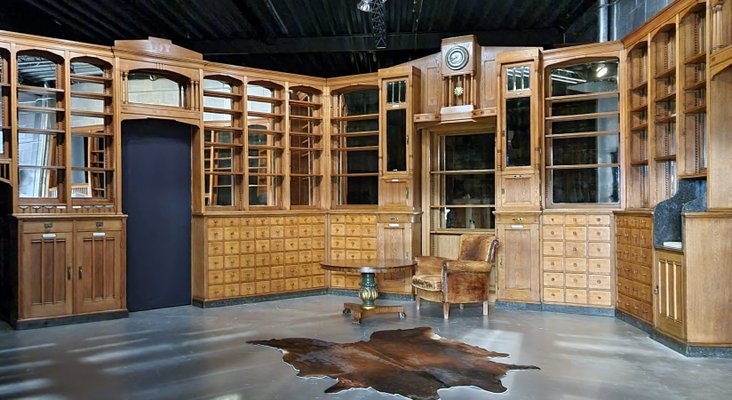The photograph presents a meticulously staged room designed to evoke the atmosphere of an opulent cigar or smoking room, but upon closer inspection, it reveals its true setting within a warehouse. The soaring black corrugated metal roof with visible black support beams and cinder block walls at the top left expose the utilitarian location. The floor is a smooth, flat concrete.

Dominating the room is an extremely ornate cabinet that spans several sections, featuring tall bookshelves with a mix of filled and empty shelves on the upper halves, extending across three walls. Below the shelving units, dark wood cabinets and lighter oak wood drawers showcase intricate craftsmanship and detailing, including a clock stationed prominently at the center. 

A striking round table anchors the room, accompanied by a plush leather armchair positioned perfectly for relaxation or reading, suggesting an environment that blends luxury with comfort. The setting is completed by a distinctive cowhide rug in the center foreground, adding a touch of rustic elegance below the polished interior.

Despite the elaborate setup, subtle cues like the industrial ceiling and walls discreetly remind viewers of the staged nature of this sophisticated display.